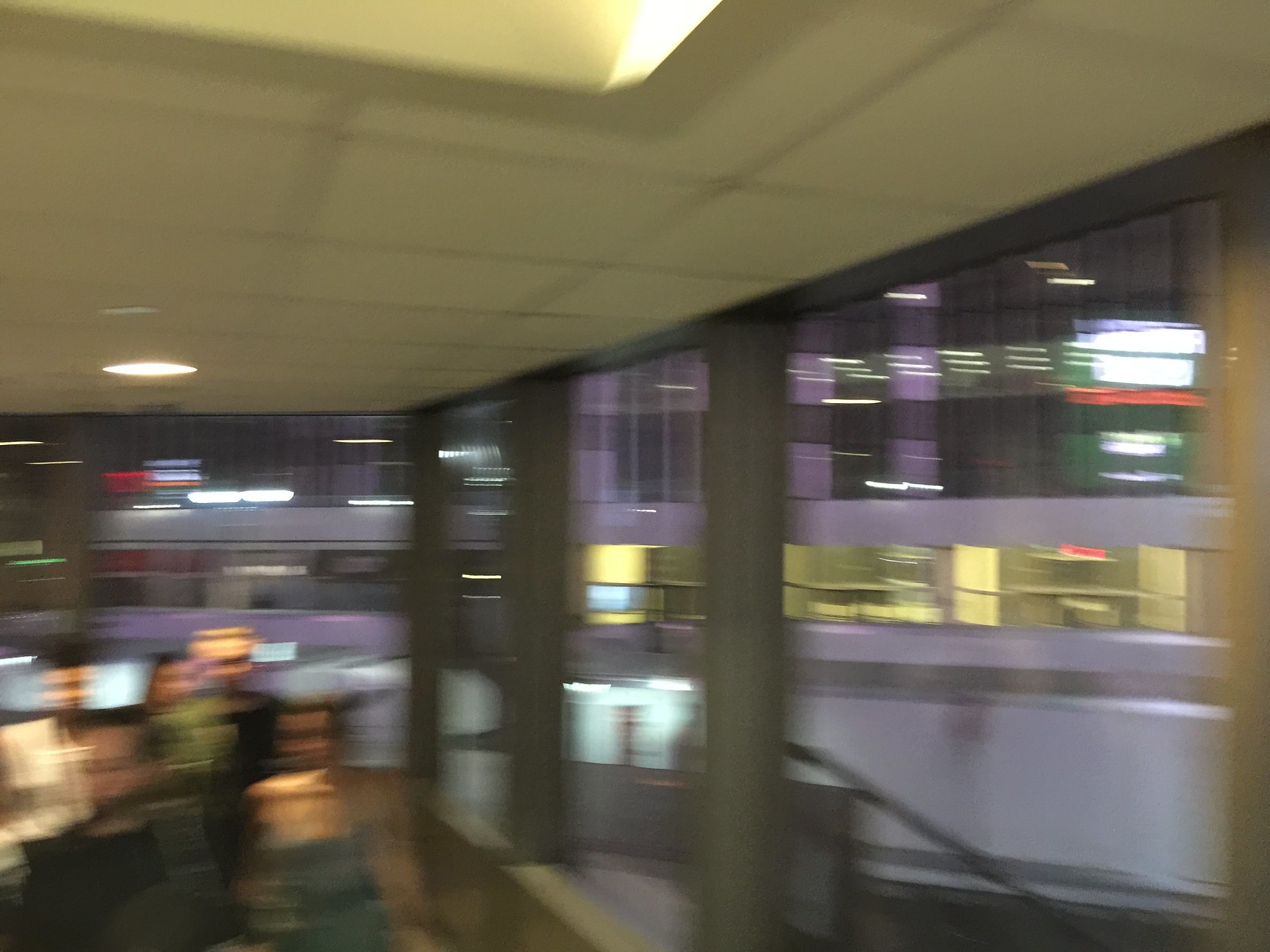This color photograph captures the blurry interior of what appears to be a retail establishment, likely a cafe or restaurant. The establishment features a yellow ceiling, which may be influenced by the interior lighting as the actual color could be grey or white, and it is adorned with tiles. A small light fixture is visible on the left side of the image. The building is surrounded by large windows through which cityscape with illuminated tall buildings can be seen. In the bottom left corner, at least four people are discernible. One man is wearing a white shirt, and beside him a woman is either wearing a green shirt or standing closely behind another individual. Additionally, a man with yellowish hair or a yellow hat is visible next to another person in a light-colored shirt, holding a dark object, further suggesting a lively dining environment.